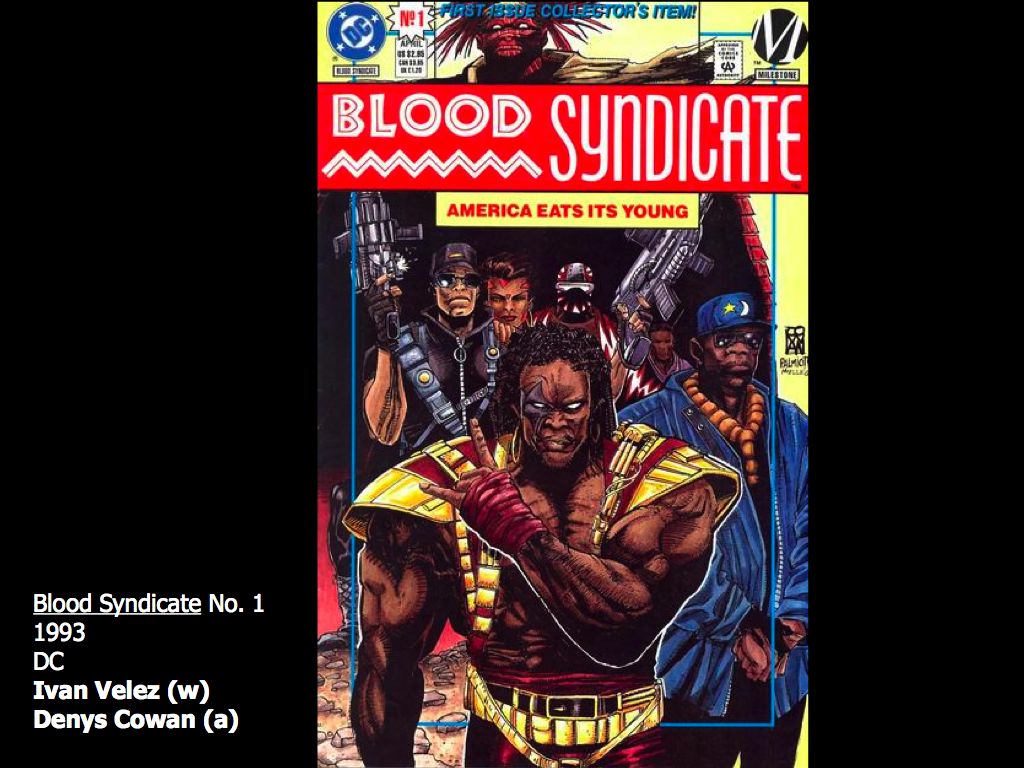The image is a detailed cover of the first issue of the comic book "Blood Syndicate," published in 1993 as part of the Milestone Initiative by DC Comics. The cover features vibrant colors, including red, yellow, blue, and various earth tones. At the top left, there's a blue circle with four white stars and the text "DC" diagonally. Adjacent to it, on the top right, is a white "M" inside a black circle. The top of the cover is dominated by a red banner with white lettering reading "Blood Syndicate," underlined by a double white zigzag. Beneath this is a yellow band with red text stating "America Eats Its Young."

The central figure on the cover is an angry-looking warrior with black skin, long braided hair, and a red face with white eyes. He wears gold shoulder armor, a large belt, and a bandage around his hand, which is positioned in front of his shoulder in a rock symbol, with the forefinger and pinky finger extended. Positioned to his right is a man in a blue baseball hat, black sunglasses, a bead necklace, and a large blue coat. He epitomizes a gangsta style appearance. In the background are several men, dressed in black gear and holding silver guns, adding to the menacing atmosphere.

At the bottom left of the cover, white text reads: "Blood Syndicate, Number 1, 1993, DC," along with the credits "Ivan Velez (W)" and "Dennis Cowan (A)." The entire cover reflects a striking comic book illustration in a portrait orientation.